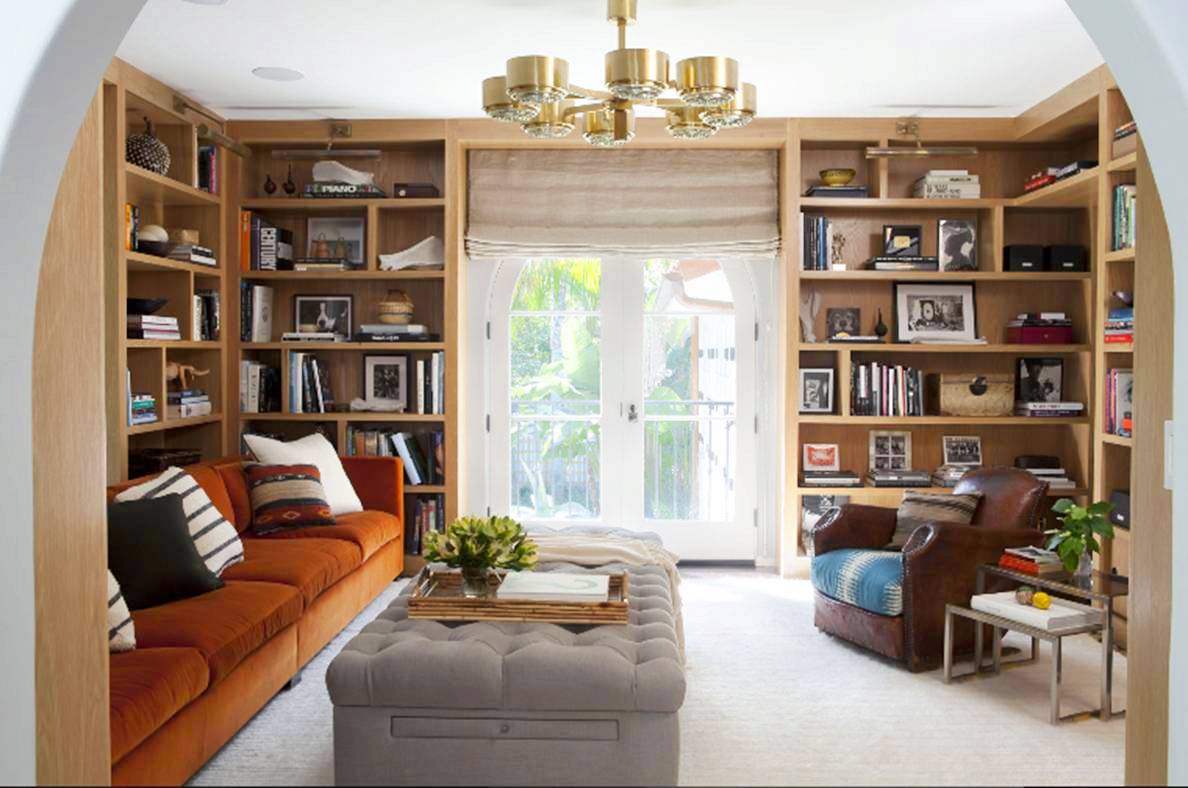This is a photograph of a beautifully decorated living room that can also serve as a study. The scene is viewed through a wide white archway, revealing an inviting space filled with wraparound bookshelves crafted from a nice light wood. On the left side, there's a long rust-colored sofa that extends from the lower front corner towards the back. Complementing this is a brown leather recliner on the right side, accompanied by a small coffee table that holds a plant and a book. Centered in the room is a gray ottoman, topped with a tray and another flowering plant. The back wall features two large patio doors opening out to what appears to be a balcony, with palm trees visible in the background. Above, a modern gold chandelier hangs from the white ceiling. The bookshelves are packed with books, picture frames, photographs, sculptures, and various mementos, adding a personal touch to the space. The room is unified by a white carpet that grounds the differing wood tones and vibrant colors.